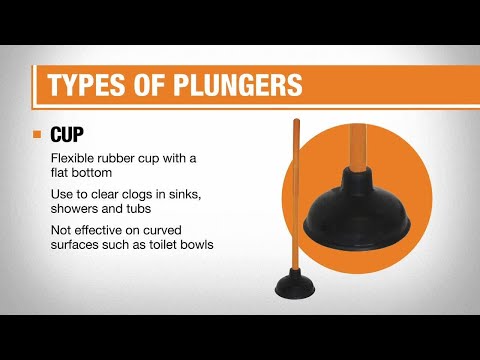The image displays an informational video screen capture about different types of plungers, with prominent details on a white background. It features a large orange rectangle at the top, containing white text that reads "Types of Plungers." Below this, on the left side, a small orange square bullet point precedes the word "Cup" in bold black letters. Accompanying this text is a detailed description in smaller black font that reads, "Flexible rubber cup with a flat bottom used to clear clogs in sinks, showers, and tubs. Not effective on curved surfaces such as toilet bowls." To the right of this description, there is a visual representation of a cup plunger. This includes a main image of a black plunger with a brown wooden handle standing upright against the frame and an adjacent orange circle highlighting a close-up view of the plunger’s rubber cup. The image serves as a clear and comprehensive introduction to a specific type of plunger, highlighting both its appearance and functional limitations.